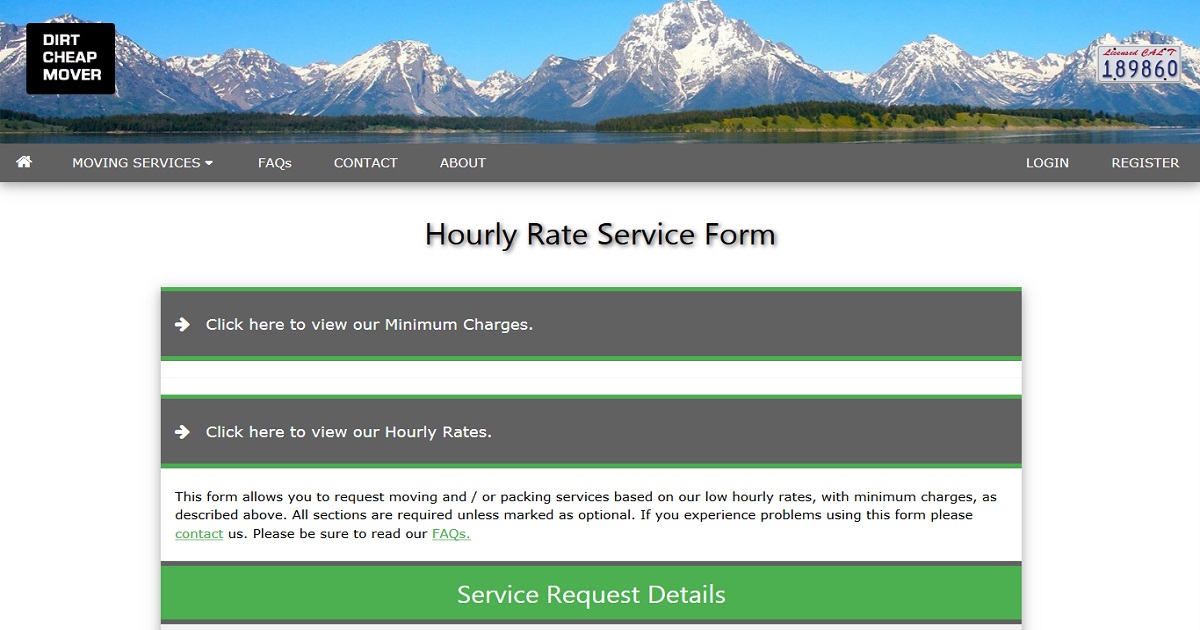Screenshot from Dirt Cheap Movers Website

The screenshot captures the homepage of Dirt Cheap Movers, featuring a prominent banner image of tall, snow-covered, rocky mountains. The top navigation menu includes options for Moving Services (with a drop-down menu), FAQs, Contact, About, Login, and Register. Below the banner, in a gray section with white text, there is a clickable link stating "click here to view our minimum charges." Another banner follows, inviting users to "click here to view our hourly rates."

A white section beneath these banners outlines the purpose of the service form, which allows users to request moving and packing services based on the company's low hourly rates and minimum charges. It clarifies that all sections of the form are required unless marked as optional. If any issues arise while using the form, users are directed to click the underlined, green-colored "Contact" link for assistance. Additionally, there is a reminder to read the FAQs, also highlighted in underlined green text.

At the bottom of this section, the heading "Service Request Details" indicates where the user can input specific information regarding their moving or packing request.